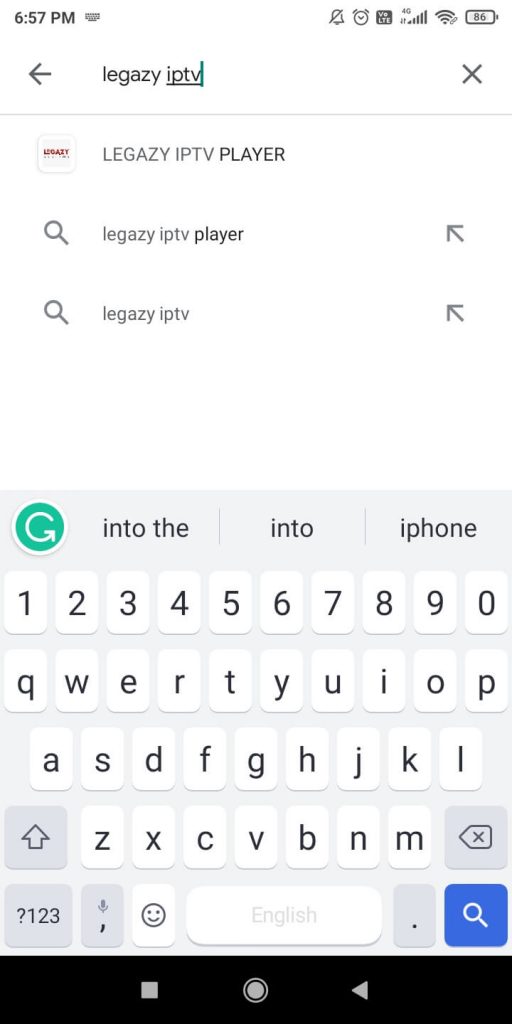A screenshot of a smartphone screen captured at 6:57 p.m. is displayed. At the top-right corner, there is an icon of a bell with a diagonal line through it, indicating 'Do Not Disturb' mode. Next to it is an alarm clock icon, followed by a small calendar icon. Four signal bars are displayed, with three of them filled in black, suggesting moderate network signal strength. The Wi-Fi signal icon follows, and the battery icon shows a charge level at approximately 55%.

Below the status bar is a search box containing the text "LEGAZY IPTV," with "IPTV" underlined. Beneath this, the text "LEGAZY IPTV player" is displayed, followed by a magnifying glass icon labeled "LEGAZY IPTV player" with an arrow pointing upwards and to the left. Next, another magnifying glass icon is labeled "LEGAZY IPTV" with an upward-left pointing arrow.

The QWERTY keyboard is open at the bottom of the screen. At the top of the keyboard, there is a circle icon with an arrow inside it, curving upwards and to the right. Text labels "INTO THE," "INTO," and "IPHONE" are displayed next to this icon. The standard keys of the keyboard are visible below these elements.